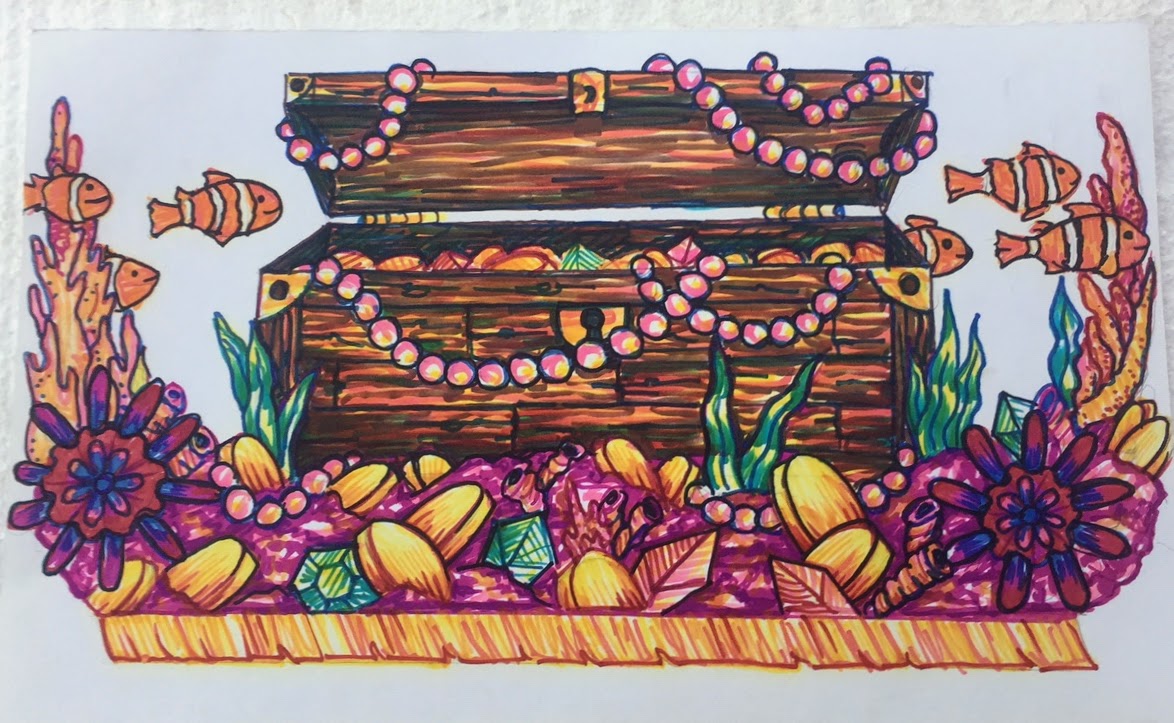In a vivid, marker-drawn underwater scene, a variety of coral and sea creatures, including several little clownfish, swim past an open treasure chest. The chest overflows with vibrant gold coins, glittering stones, and delicate strands of pearls, all rendered in striking, eye-catching marker colors. The artist has chosen a whimsical, non-realistic style, evident in the playful bleeding of ink, such as where the orange and black markings of the clownfish merge. The scene focuses solely on the treasure chest and its immediate surroundings, with no depiction of water or underwater effects. Everything is set against the stark contrast of plain white paper, emphasizing the richness and liveliness of the illustrated treasures and marine life.